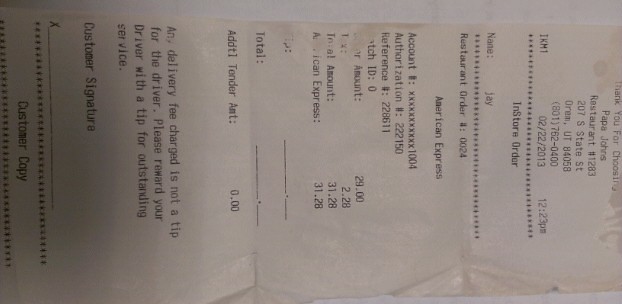A receipt from a Papa John's restaurant in Utah is prominently featured in this image. The receipt is positioned sideways, with the top facing to the right, and it rests on a plain white background. This white paper receipt, displaying black text, shows slight signs of wear, evident through minor folds and wrinkles. Despite some fading and discoloration in the print, the details remain legible. The total amount of the purchase is $31.28. The transaction was handled by a cashier named Jay and was paid using American Express. The in-store order was placed at precisely 12:23 p.m. on February 2, 2013.